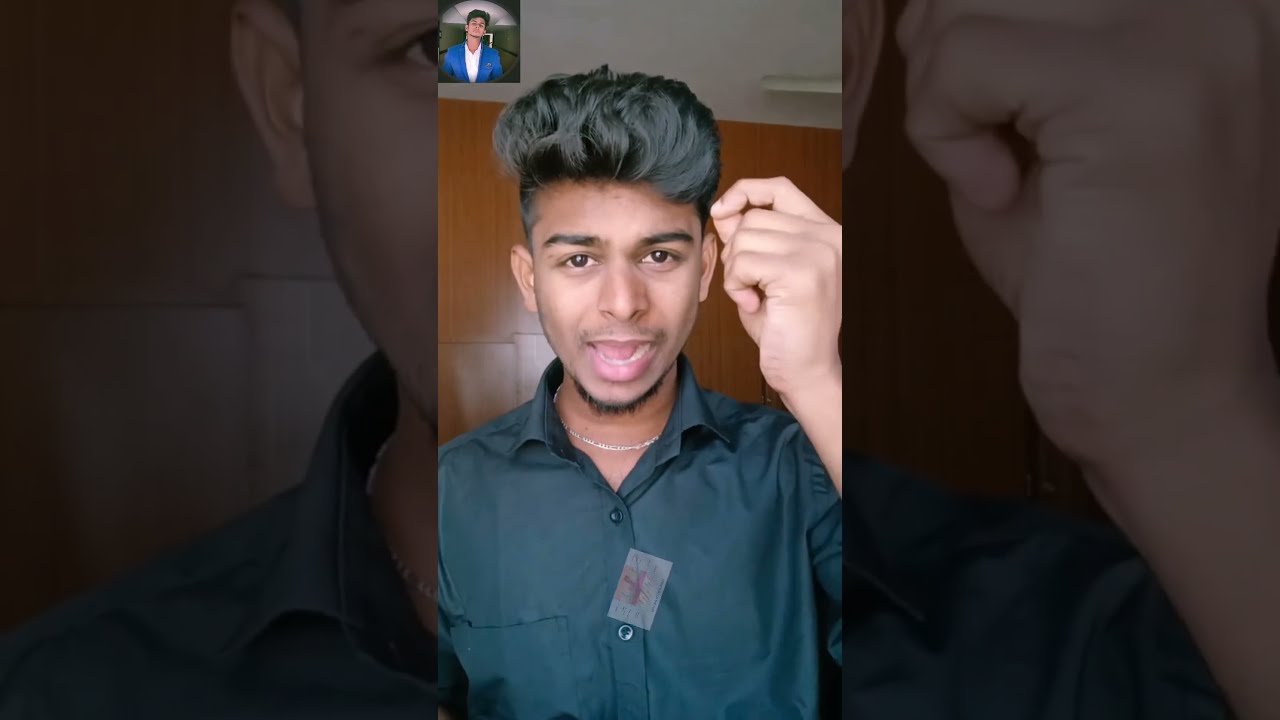This is a detailed rectangular photograph showing a young man with short black hair styled upwards, approximately two inches long. He has thick black eyebrows and a small goatee with sparse mustache hairs. The young man is wearing a dark greenish-gray button-down collared shirt and a silver necklace. His mouth is open, revealing his tongue and teeth, giving an impression of either speaking or reacting, possibly saying "ouch," as he has his left hand raised towards his forehead, appearing to pull out a single hair.

The background features a wooden wall, with a white ceiling above. In the upper left-hand corner of the image, there is a small inset showing another man, dressed in a blue suit jacket and white dress shirt, possibly indicating a video call or similar scenario. The overall composition includes additional vertical rectangular sections that offer close-ups of the young man's face and his hand, enhancing the focus on his expressive action.